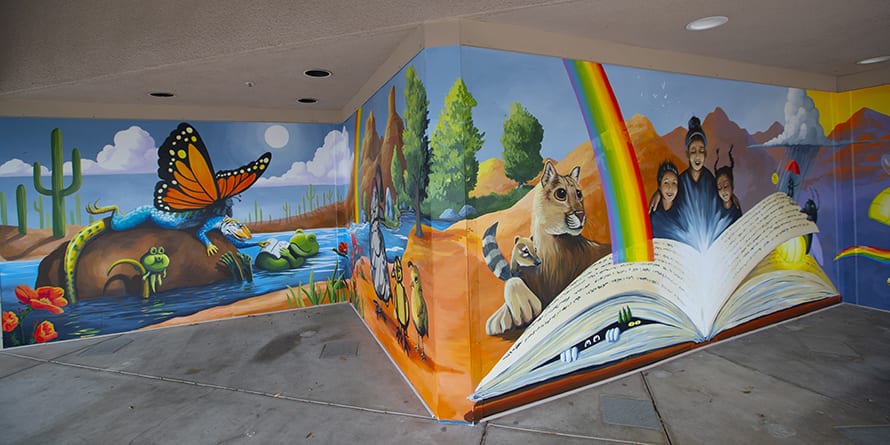This vibrant color photograph captures an intricate and expansive mural adorning the interior walls of a building, possibly an exhibit, school, or library. The setting features a gray concrete floor and ceiling with recessed lights, two of which are illuminated, enhancing the mural’s rich hues. The walls showcase a strikingly colorful scene with a large book from which a rainbow emerges, creating a focal point that holds the gaze. Positioned around the book are various animals and figures: a black and white mountain lion, a raccoon perched on its paw, and three women with a look of contemplation. Beside these, a butterfly with orange monarch wings rests atop a lizard above a brown animal submerged in water, with a frog perched on its back. The background of the mural is teeming with additional natural elements, including flowers, clouds, cacti, mountains, and trees, all rendered in vivid blues, yellows, and reds. This beautifully detailed mural turns the entire space into a colorful tapestry of nature, storytelling, and imagination.